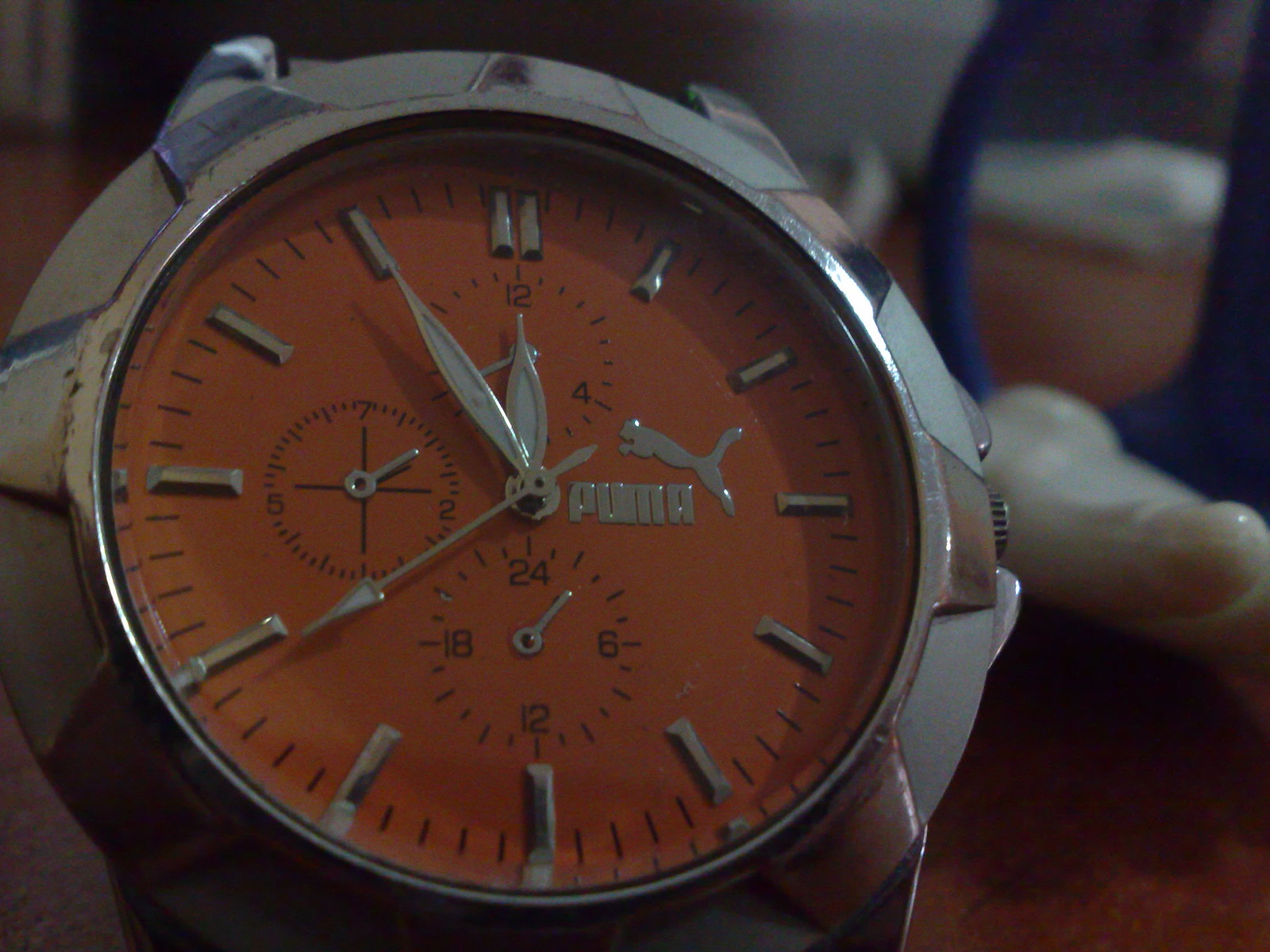In the image, the backdrop is predominantly dark, creating a subdued atmosphere. Amidst this, a translucent blue circle offers a view of a brown table surface. On this table, a person's fingers or toes are slightly visible, hinting at human presence. The central focus is an antique wristwatch resting on the table. The watch, with its silver casing, exhibits signs of age, including some rusty spots marring its once pristine surface. The watch face is a faded orange, marked only with minimalist silver lines in place of numerals and silver hands for timekeeping. The brand name "Puma" is prominently displayed in silver, accompanied by an emblematic silver puma figure, adding a touch of elegance to the vintage piece.